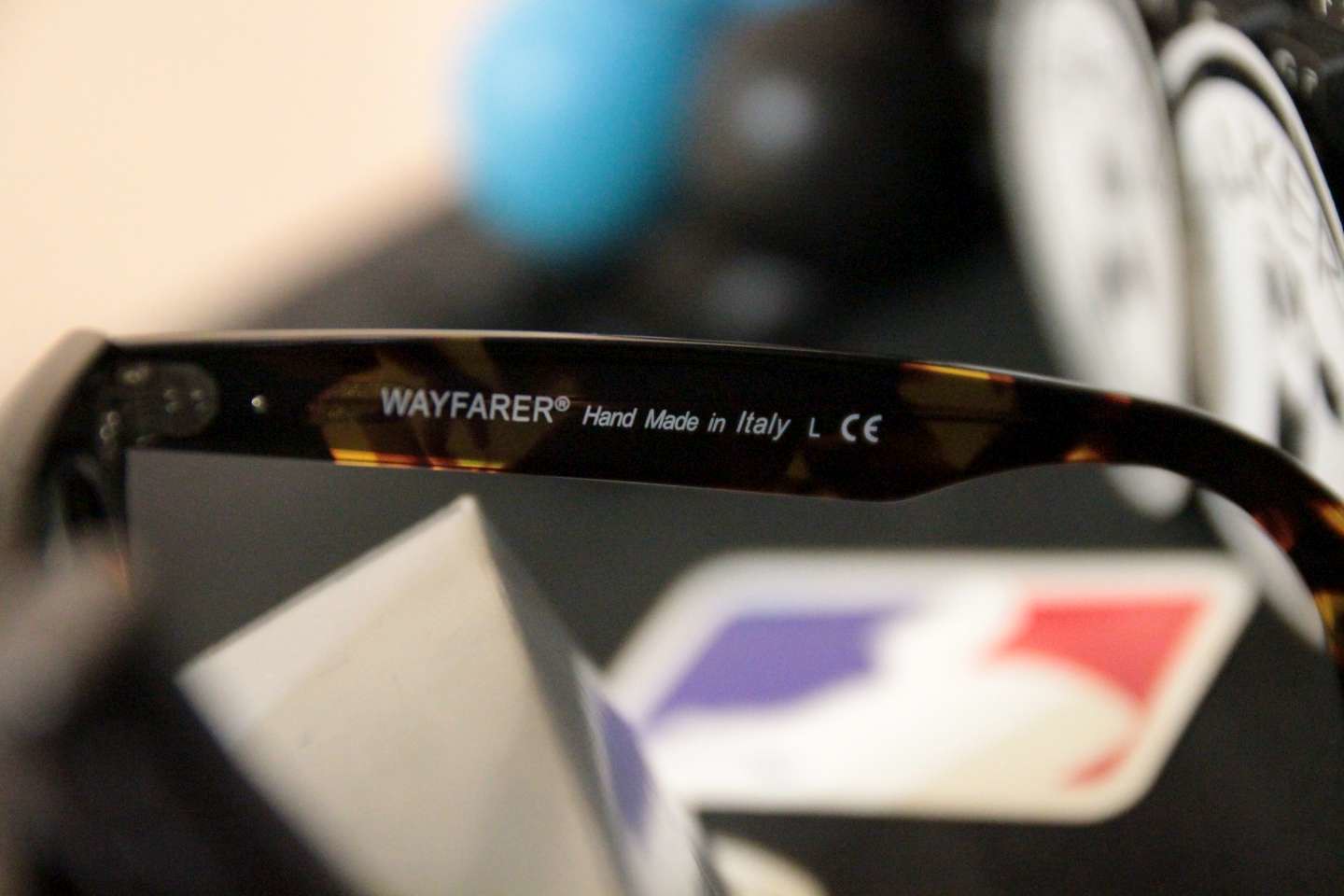This color photograph features a prominently blurred background, presenting objects in hues of black, blue, white, and an indistinct blue and white icon. Among these, a specific object stands out in the foreground: a pair of sunglasses, or more precisely, the arm of the sunglasses which is designed in tortoiseshell plastic. The arm showcases detailed white capital letters reading "WAY FARER." Below that, in smaller text, it states "HAND MADE IN ITALY," followed by the letters L, C, and E. The photograph captures the sunglasses as the central focus, perfectly framed against the slightly blurred, possibly indoor background, suggesting an ordinary setting like someone's home or a retail store. The blend of colors including black, white, off-white, light blue, gray, red, and purple adds to the elegance and casual complexity of the scene.